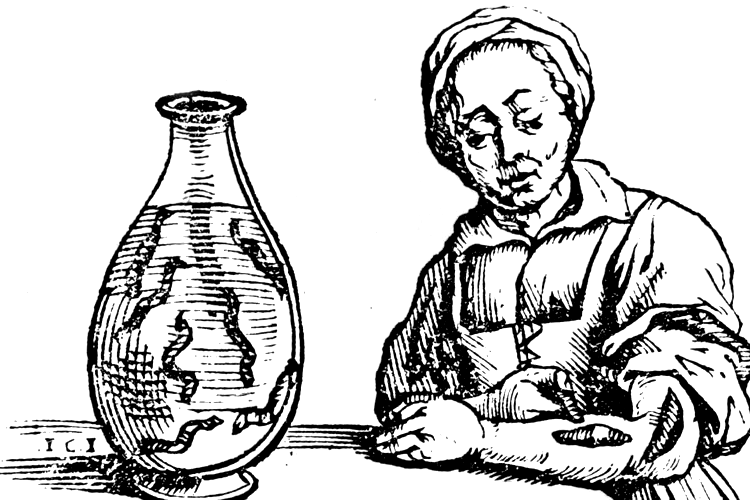This detailed ink illustration on a white background depicts an older woman, likely in her 50s or 60s, engaging in a historical medical practice using leeches. She is dressed in an old-time, collared blouse with long sleeves, the right one rolled up above her elbow, and a pinafore or apron over it. Her head is wrapped in a cloth, allowing a bit of hair to peek out. Positioned on the right side of the image, the woman sits at a table located to her left, her hand resting on it. 

On her exposed forearm, several leeches are visible; two are already attached, and she appears to be placing a third one. Adjacent to her on the table, there is a large glass bottle with an oval base that narrows at the top, resembling a vase. The bottle is three-quarters filled with fluid, in which seven more leeches can be seen. This scene vividly illustrates the historical use of leeches in medical treatment to draw blood. In the lower right corner of the image, some indistinct and slightly blurred letters can be observed, possibly reading "ICI" or "YCX."